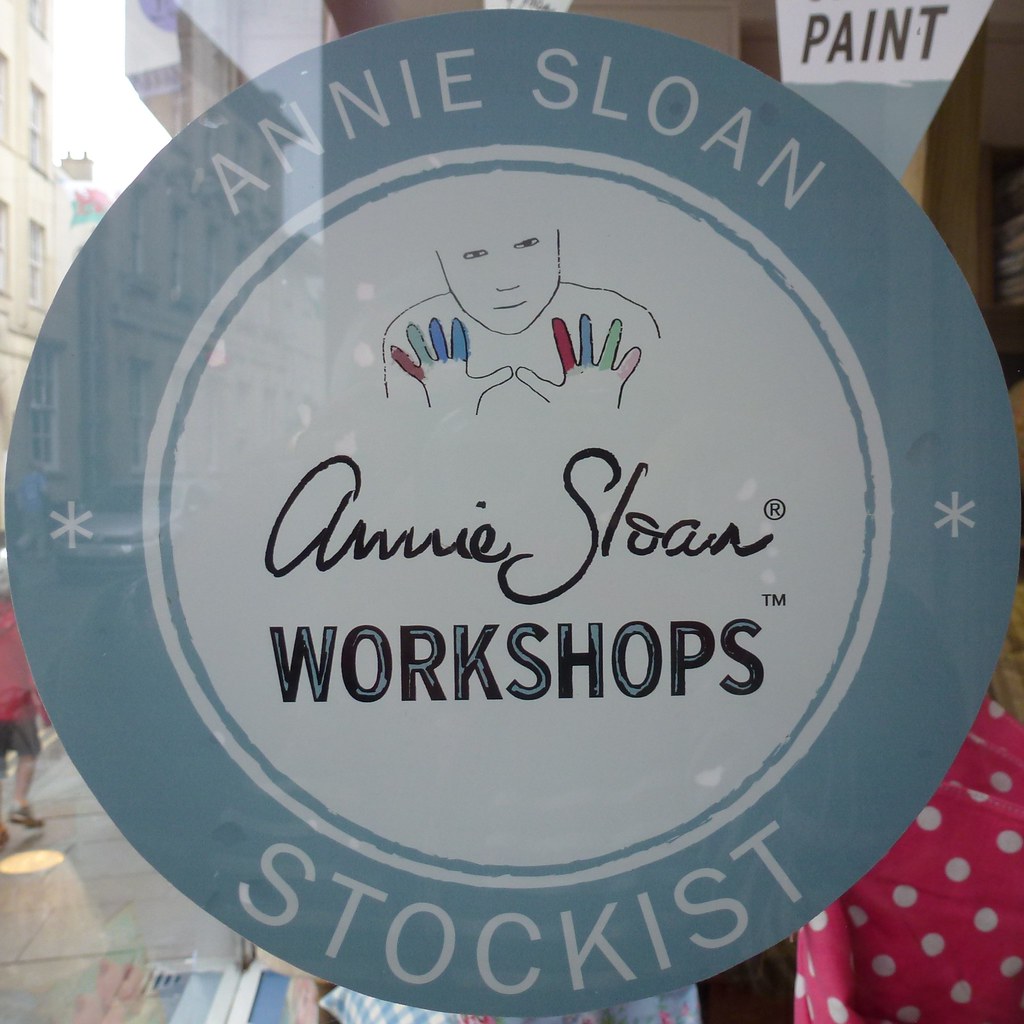The photograph captures a shop window with a prominent circular logo adhered to the glass surface. The round symbol has a light blue border and a white inner circle. Along the top edge of the blue border, "Annie Sloan" is written in white letters, while the bottom part features "Stockist" in a similar white font. Within the central white circle, the logo showcases a sketch-like silhouette of a person with two raised hands, each finger painted differently in vivid colors like green, blue, light blue, red, dark red, and pink. Above the figure, “Annie Sloan” is inscribed in a signature font, with "Workshops" in black and gray letters below. Adorning the sides of the logo are small snowflake motifs. Reflections on the glass reveal beige old city buildings, a sidewalk, and a person walking by in red shoes, brown shorts, and a red hoodie. Additionally, the upper right corner of the window displays another sign with "paint" in black letters.